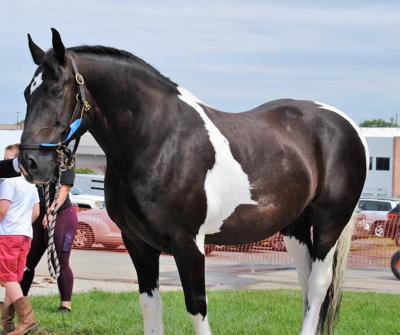This is a small square image featuring a Pinto horse, primarily dark brown with several distinctive white markings: a zigzag stripe on its midsection, white patches on its hindquarters, and a white patch on its forehead. Its legs are dark brown down to the knees, transitioning to white down to the hooves, while the hind legs are mostly white. The horse's mane is almost black, and its tail is a mix of light brown and white. It wears a black and blue harness, with a gray and black rope attached.

In the background, there is an overcast sky filled with layers of white and gray clouds. The horse stands on a grassy area, with a parking lot visible behind it, separated by an orange netted fence. Several people are walking nearby: a man in a white t-shirt, red or peach-colored shorts, and brown boots, and a woman who appears to be wearing dark leggings, possibly maroon pants, and a black shirt. The overall setting suggests it might be a horse show, as the horse appears to be posing for the picture.